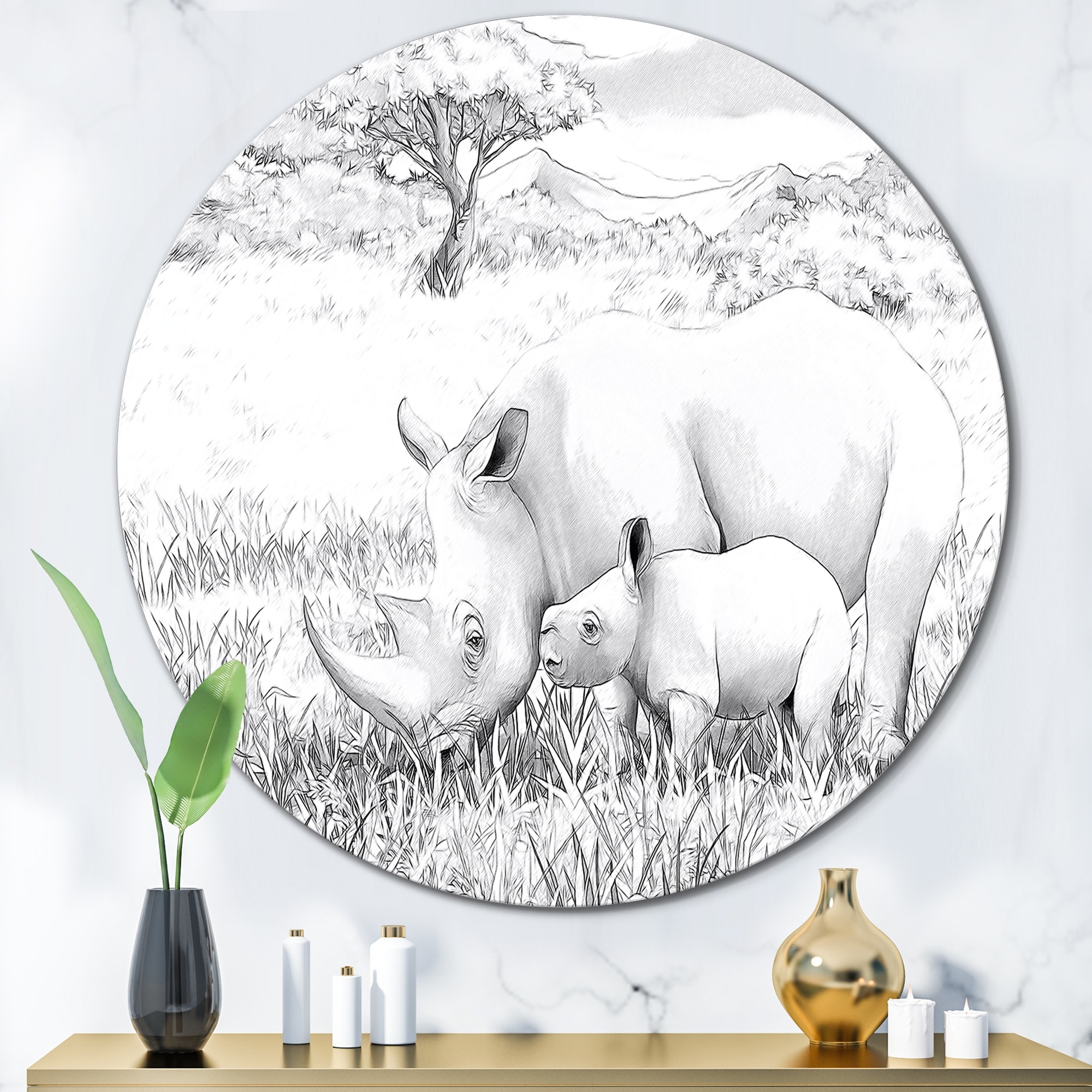The CGI design image depicts a striking circular black-and-white painting fixed on a marble-like wall. The artwork features a mother rhinoceros centrally positioned, looking down to graze on some grass, with a baby rhino nestled directly underneath, nuzzling the mother's head. The backdrop of the scene presents a serene landscape with a mountain range, a single prominent tree, and a few scattered bushes, enhancing the sense of a natural savannah.

Below this engaging artwork, a table is set with tastefully arranged items. On the right, there are two white candles and a gold vase with a distinctive bulge. To the left, there are a few white bottles with gold tops, and a sleek black vase holding two light green plant leaves. The overall setting creates an elegant and cohesive visual experience, combining both artistic and natural elements.